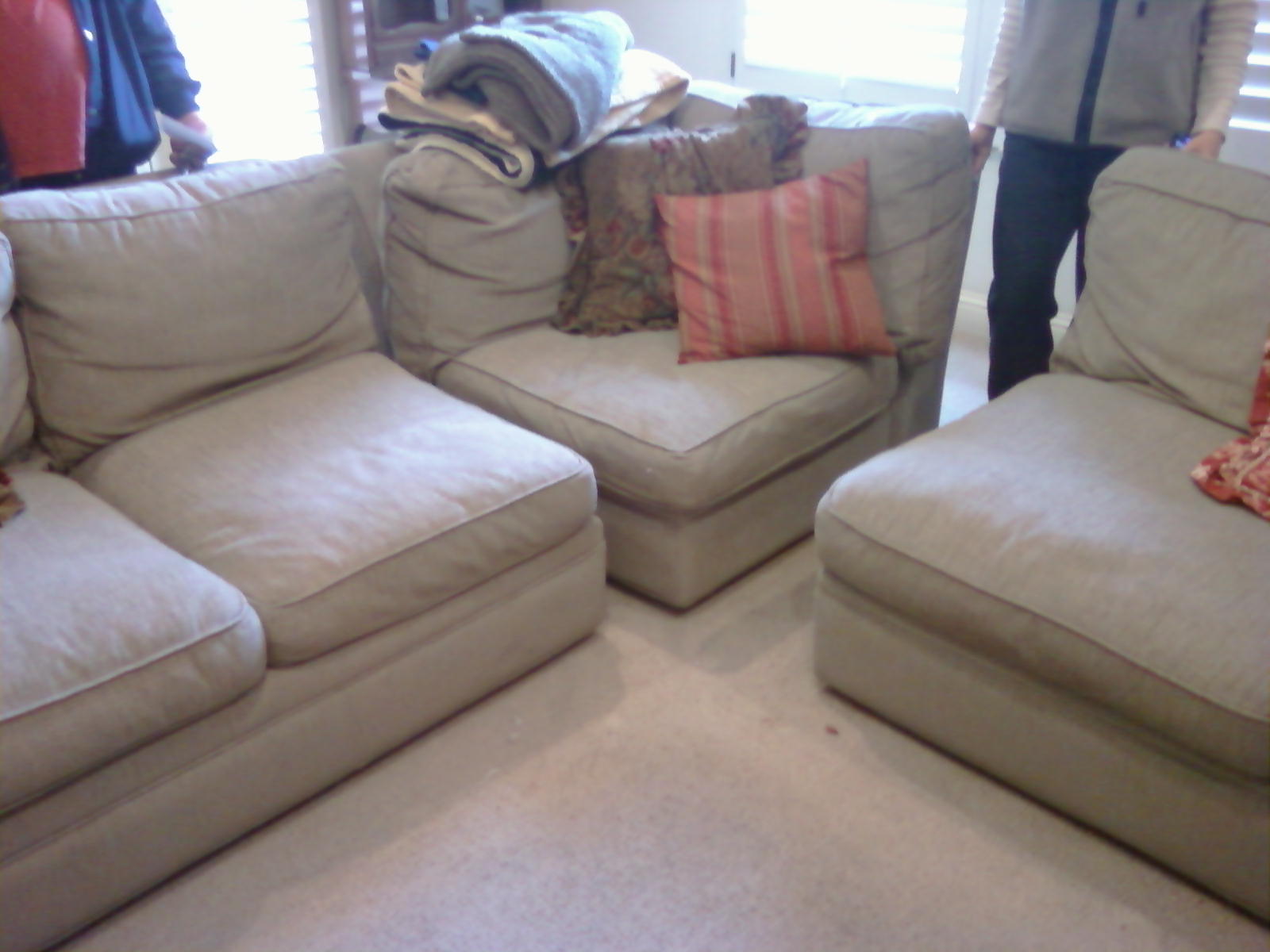The digital photo captures a daytime interior scene of a home, featuring a carpeted or possibly tile floor. In the foreground, there is a gray sectional couch with visible gaps between some sections. The couch is adorned with various pillows and blankets: a pink pillow with more pink stripes on the corner section, gray pillows, and additional blankets in shades of cream and gray. A red fitted sheet is stretched over part of the carpet and appears somewhat dirty.

On the top left of the image, a hefty individual stands behind the couch, wearing a blue jacket over an orangish-red or pink shirt, and holding a piece of paper in their left hand. On the top right, another person, dressed in a gray jacket or sweatshirt with black vertical lines and black pants, holds a phone in their left hand. This person is also described as having white skin.

The background features two bright windows letting in a lot of natural white light, illuminating the scene. Between the two individuals, a wall is partially obscured by piles of blankets on the couch. The overall setting is a mix of domestic comfort and mild disarray, suggesting ongoing activities or preparations.